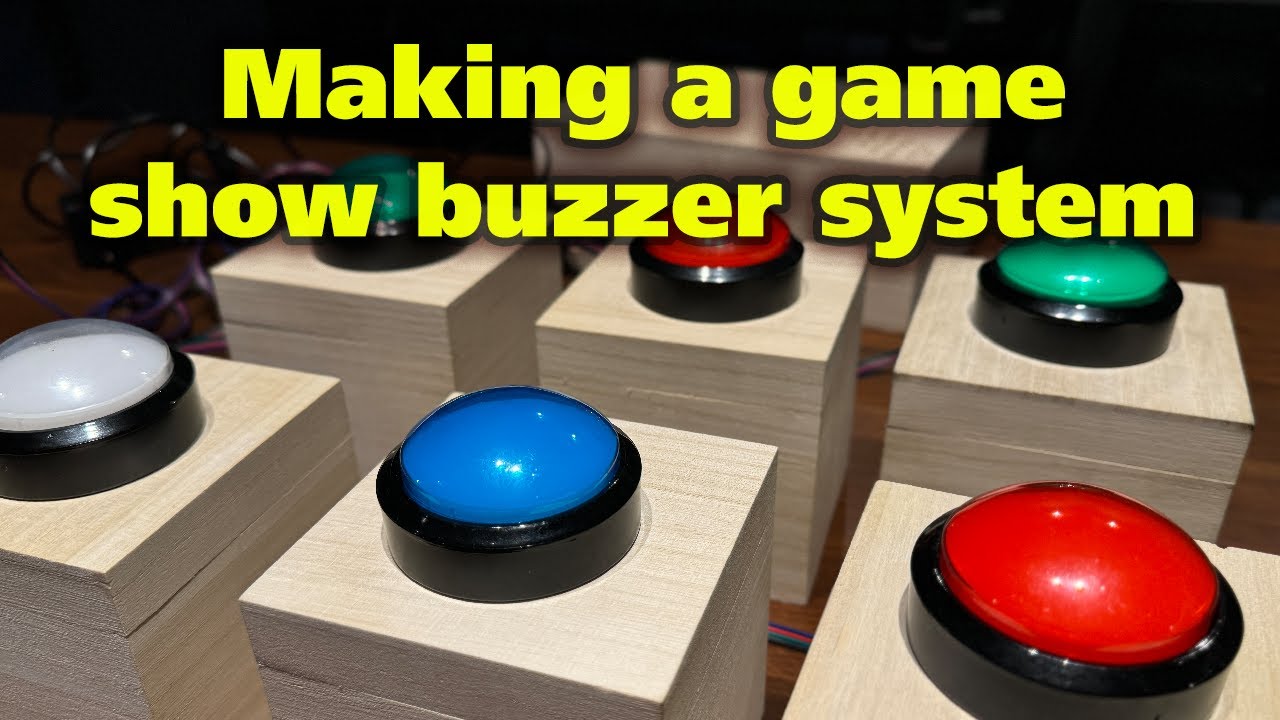This photograph features a game show buzzer system prominently displayed against a dark background. The yellow text at the top reads, "Making a Game Show Buzzer System," with a semi-transparent outline enhancing its visibility. The system comprises six large push-button buzzers, each with a black plastic base and a dome-shaped, reflective plastic top in various colors. Arranged in two rows on a square wooden cube about nine inches tall and six inches on each side, the buzzers are organized as follows: the first row from left to right has white, blue, and red buttons, while the second row has green, red, and green buttons. The setup is indicative of a game show environment, complete with visible wiring likely connecting the buzzers to the system, perfect for answering questions or pausing gameplay.